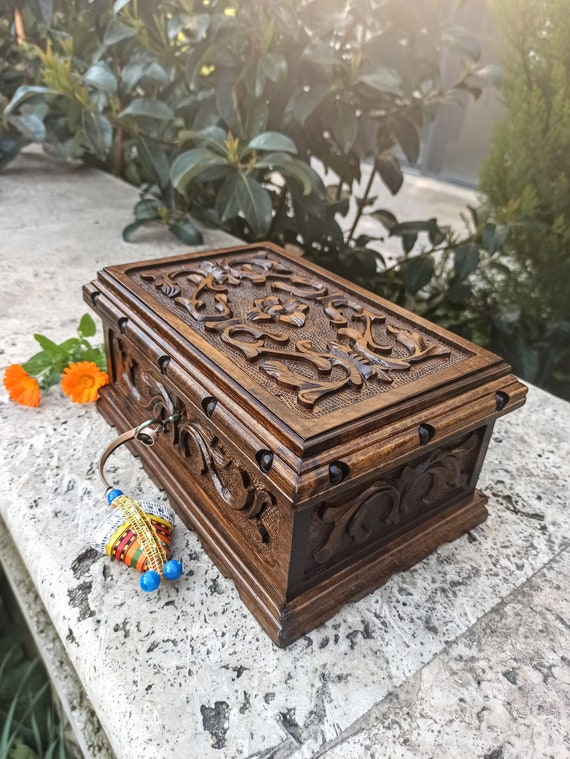This image captures a beautifully ornate oak wooden box with intricate carvings on its lid and sides, featuring leaf-like decorations and other designs. The top rim of the lid includes additional carvings, possibly resembling balls. The box sits securely on a concrete barrier, possibly a bench or fence, surrounded by lush greenery and dark green leaves. In front of the box is a triangular decorative object adorned with two blue beads. The box has a keyhole with a key, and a molded base embellished with more carvings. Orange flowers, likely daffodils, with green stems and leaves rest near the upper left corner of the box. The image might depict a grave site, but it lacks further identifying context due to the tight crop around the box.